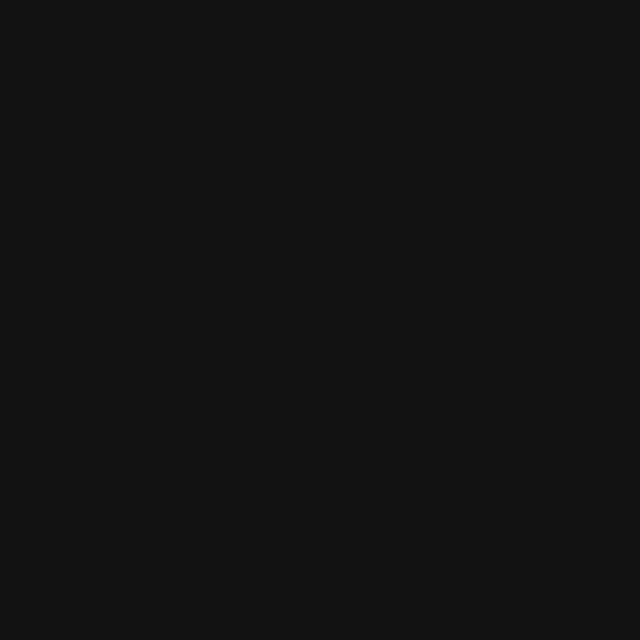A completely black webpage fills the entire frame, displaying no text, design elements, borders, or sections. The deep, solid color creates a stark and uniform appearance without any variation or details. The image presents a minimalist and unadorned black screen, devoid of any visual features or content.